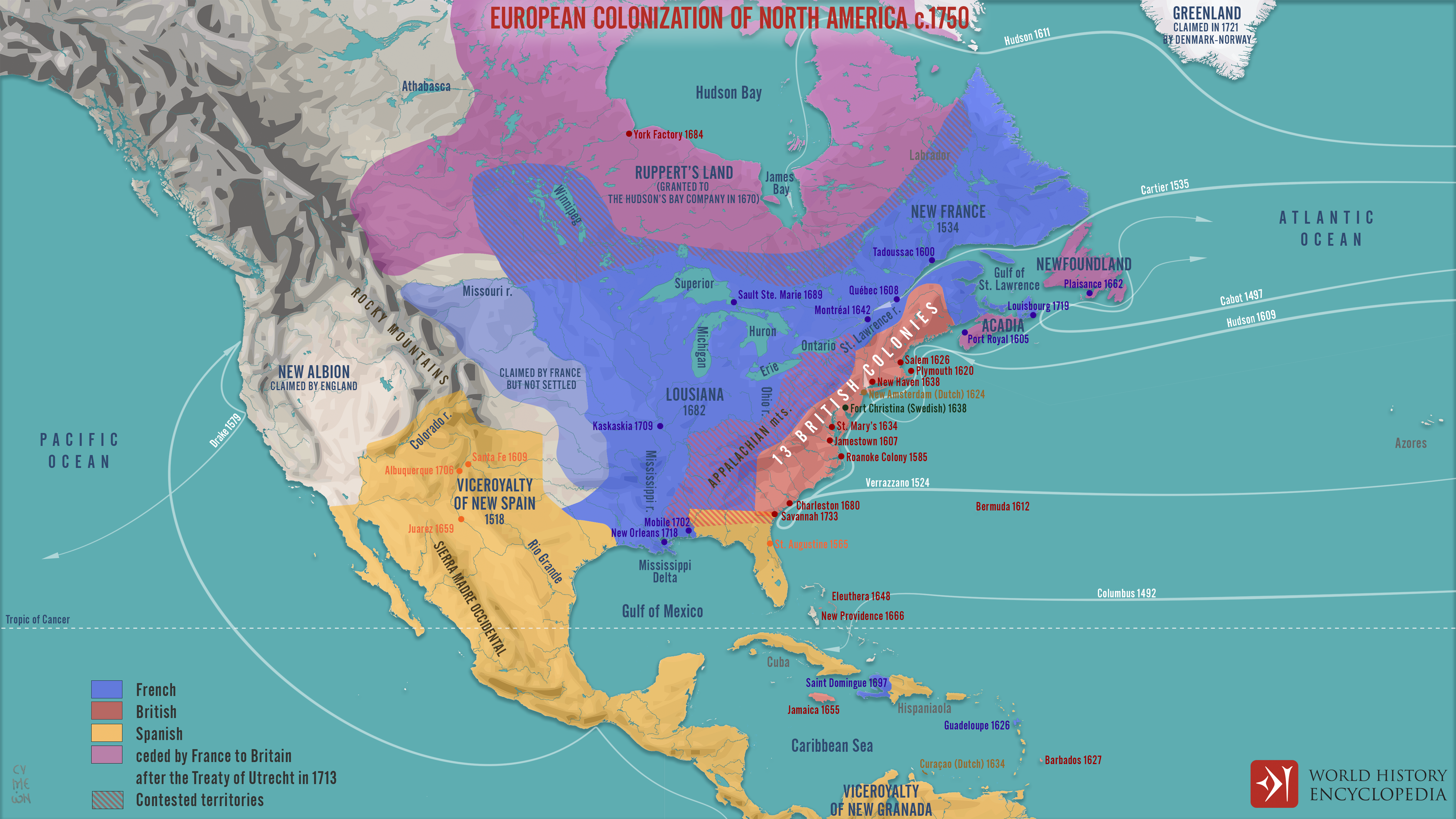This is an image of a detailed historical map titled "European Colonization of North America, c. 1750." The map's background features a blue ocean, illustrating the Atlantic, Pacific, Gulf of Mexico, and Caribbean Sea. It includes prominent labels such as Hudson Bay, the Gulf of Mexico, and Louisiana, with major features like the Tropic of Cancer line and various explorer shipping routes. The map is color-coded: blue for French territories, red for British, yellow for Spanish, and pink for regions ceded by France to Britain after the Treaty of Utrecht in 1713. Diagonal shading indicates contested territories. At the bottom, there's a burgundy and white logo beside the phrase "World History Encyclopedia." The map not only highlights territorial claims as of 1750 but also marks the year certain regions were claimed, such as Greenland in 1721 by Denmark-Norway.